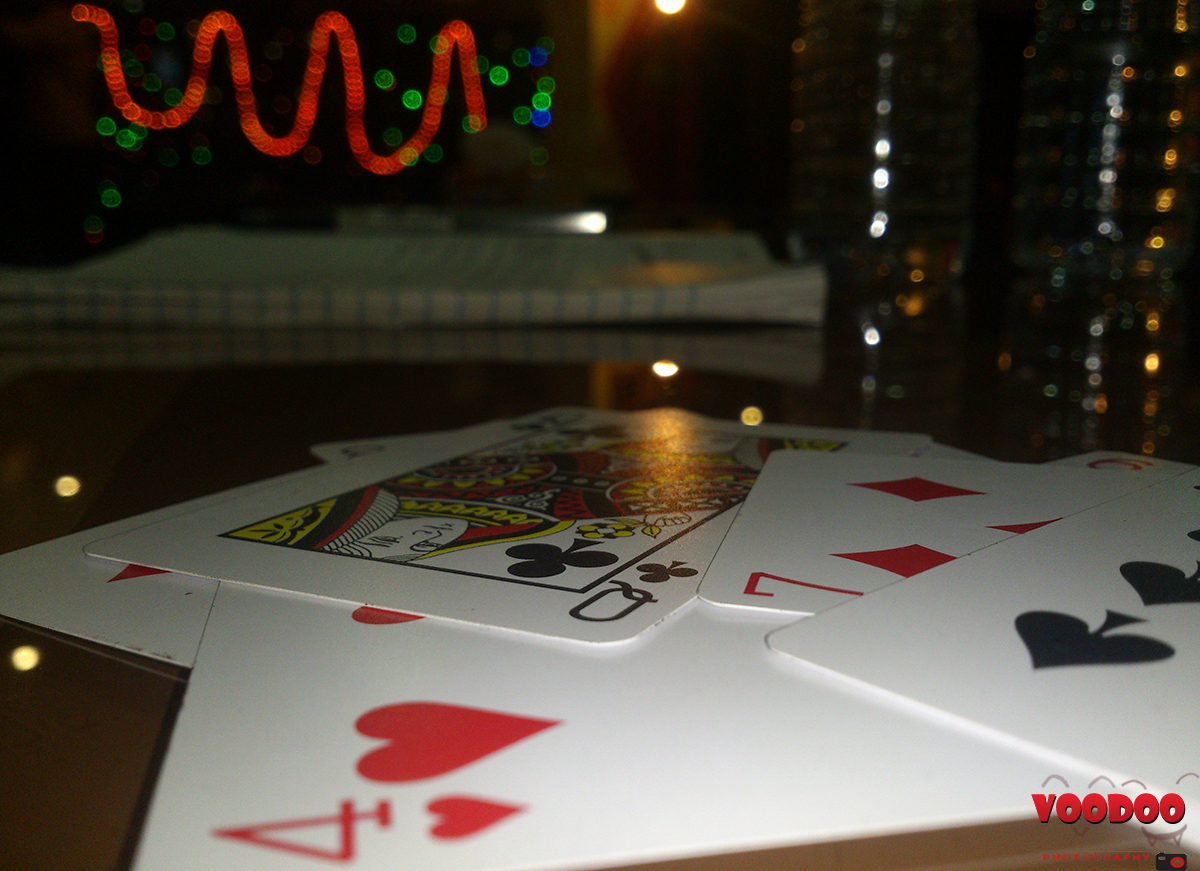This indoor nighttime photograph captures a scattered arrangement of playing cards atop a brown surface, possibly a table. The haphazardly placed cards from a standard white-background deck include the Queen of Clubs, the Seven of Diamonds, the Ace of Spades, and the Four of Hearts, overlapping each other casually. In the bottom right corner, "Voodoo Photography" is inscribed in red font; the 'O's in 'Voodoo' feature playful monster faces, complete with eyebrows, a smiling expression on the left, and a smile with vampire teeth on the right. Below this text is a small black camera logo with a distinctive red lens. The background reveals an open notebook with college-ruled paper lying flat on the surface. A series of colorful lights create a whimsical ambiance: red string lights zigzag across the wall in the upper left, interspersed with green, blue, white, and yellowish lights scattered throughout the scene.